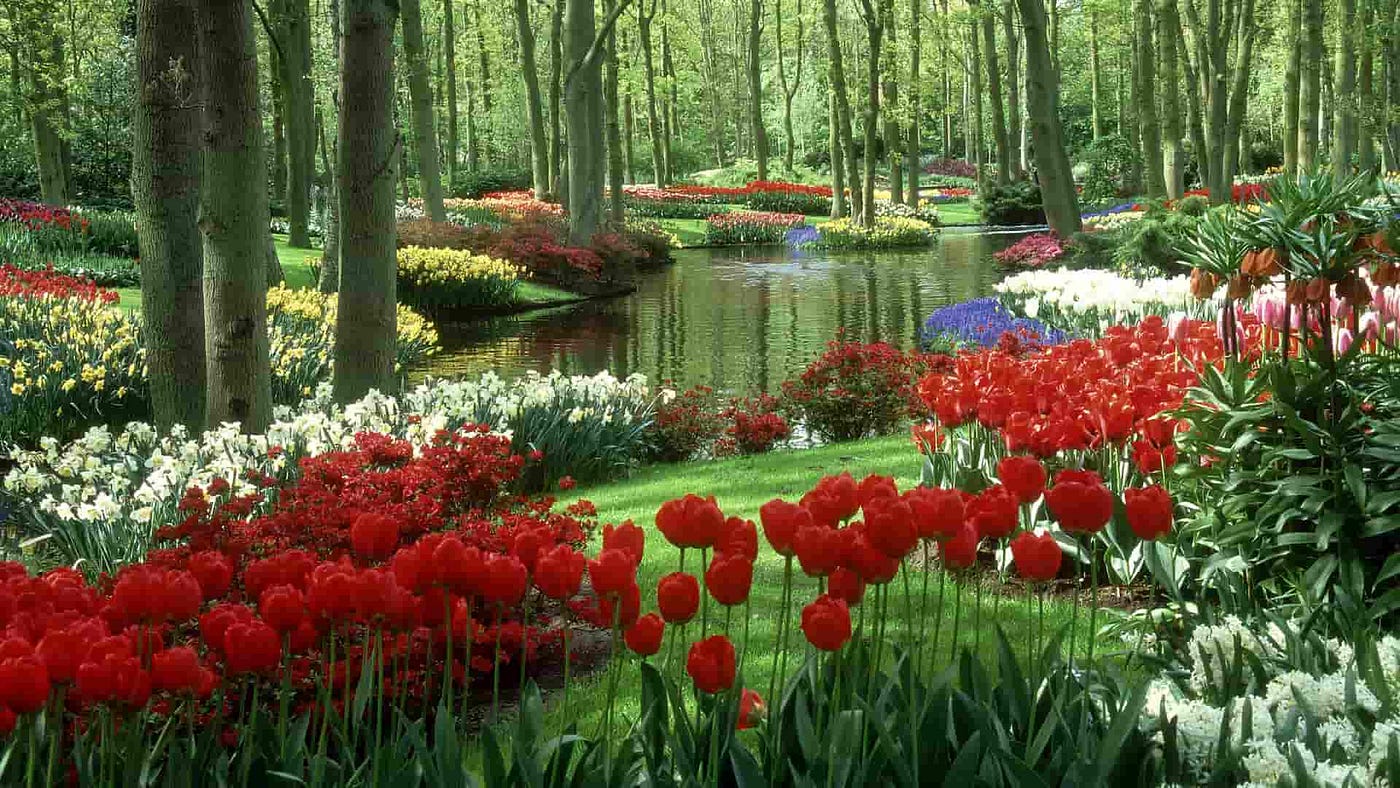This captivating landscape photograph showcases a lush, dense garden set within a wooded area, brimming with an array of vibrant flowers and greenery. In the foreground, red roses with long stems and pointed green leaves dominate the scene, accompanied by delicate white baby's breath and other fluffy white flowers. Interspersed among these are numerous varieties of flowers in blue, yellow, pink, and deep red hues. The garden is punctuated by a pond or small lake running from the left to the right, its surface adorned with ripples and lily pads, adding a serene touch to the dynamic composition. The trees encircling the garden create a dense canopy, casting both brightness and shadow, giving the area a mixture of light and dark tones reminiscent of a well-manicured swampland. The abundance of greenery, with pointy-leaved plants and stalks bearing green leaves and small brown flowers, enhances the overall lushness and vibrant atmosphere of this exquisitely natural scene.